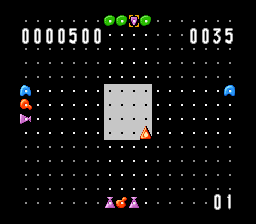The image appears to be a screenshot from a retro-style, dot-based video game. The primary display is a nearly square, slightly rectangular grid set against a black background. This grid consists of dark gray and lighter gray dots, with a central block of highlighted lighter gray dots featuring black dots within it. 

In the bottom right corner of the grid, there is an upward-pointing orange triangle with a yellow dot at its center. The leftmost side of the grid displays three icons near the center edge: a purple triangle, a red blob, and another purple triangle. 

Mirroring the left side, the rightmost side features a single blue blob aligned parallel to the blue blob on the left. Directly beneath the central block of lighter-colored dots, there are also a purple triangle, a red blob, and another purple triangle, maintaining the symmetrical theme.

The top edge of the grid holds two green blobs, a purple icon highlighted in gold, and another green icon, suggesting some form of status indicators or power-ups. 

Text indicators on the display include "000500" at the top left (possibly representing a score), "0035" at the top right (perhaps indicating time), and "01" at the bottom right (potentially a life counter). The image overall echoes classic arcade aesthetics with its simplistic yet distinct color use and symbolic icons.